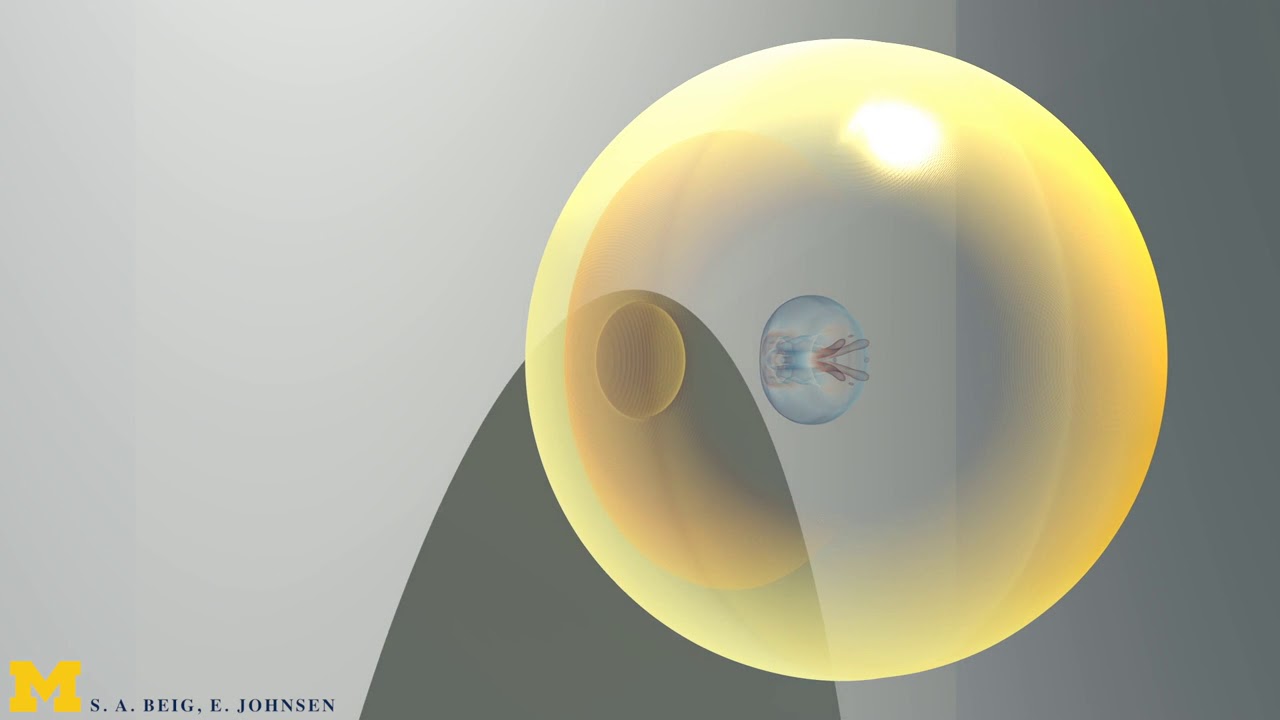The image features a gray background with three distinct shades; the left side being a lighter gray, the center a darker gray that doesn't extend all the way to the top, resembling the shape of the top of a surfboard, and the right side a medium gray. Positioned slightly off-center to the right, there is a large, translucent yellow ball displaying multiple shades of yellow. Within this yellow ball, there is a circular area on the left side shaded a darker yellow, and at the center, a blue design with intricate patterns is visible. Inside the ball, a jellyfish-like object can be seen with clear and slightly reddish protrusions. In the lower left corner of the image, the letters S-A-B-E-I-G-B and the name E. Johnson are inscribed, alongside a prominent yellow 'M' suggesting a connection to the University of Michigan.